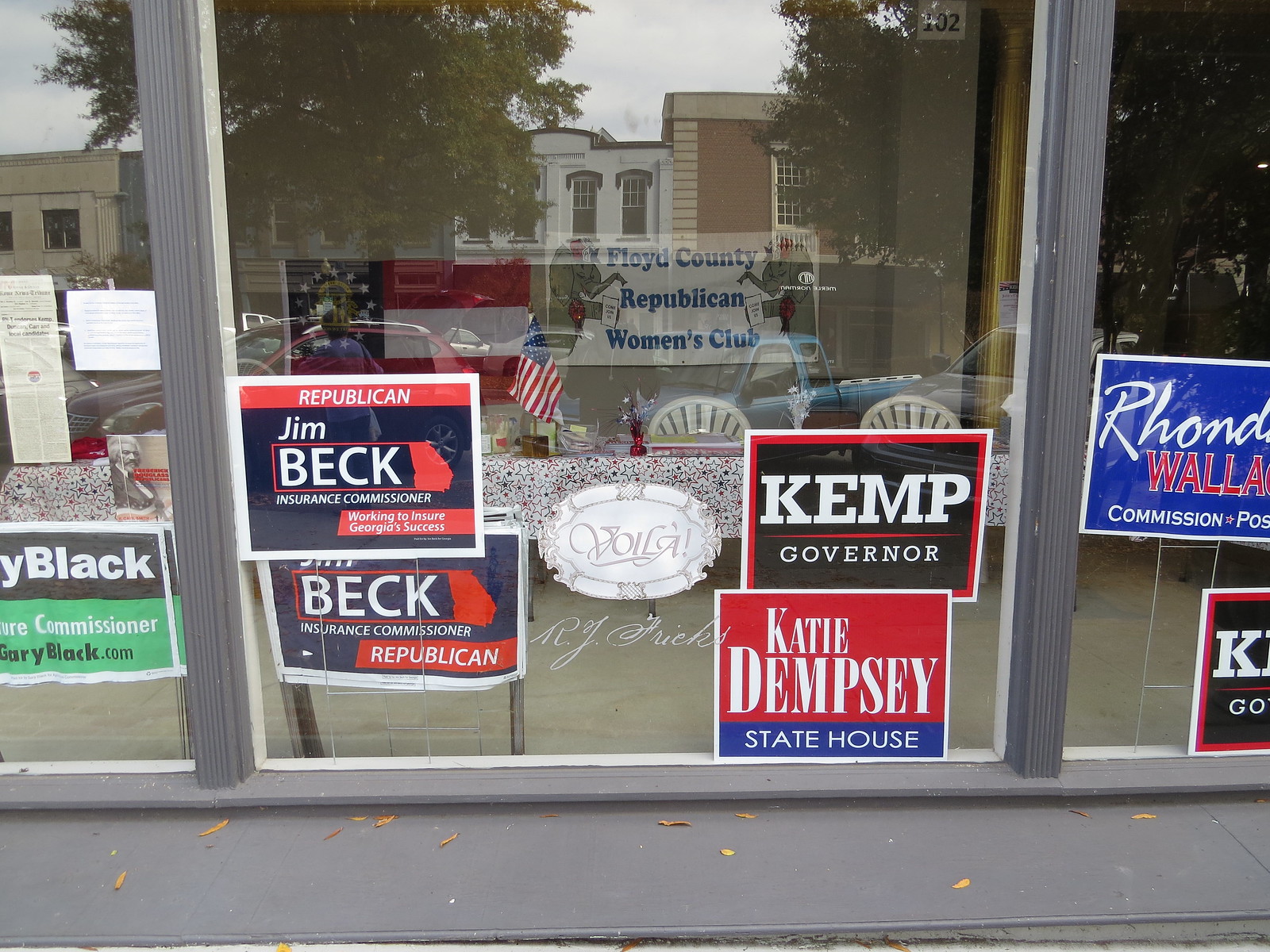This photograph captures the exterior of a gray building's window front along a sidewalk. The large, transparent windows, framed in gray, display a multitude of political campaign posters. Prominently featured are signs advocating for Republican Jim Beck for Insurance Commissioner, Kemp for Governor, Katie Dempsey for Statehouse, and Rhonda Wallace for Commission, although some of these posters appear partially cut off. Through the clear windows, the interior reveals a room set up with a folding table draped in a black-and-white starred tablecloth, positioned with chairs facing the window. An American flag is placed on the table, contributing to the patriotic decor. On the wall inside, a sign reads "Floyd County Republican Women's Club," emphasizing the political theme of the establishment.